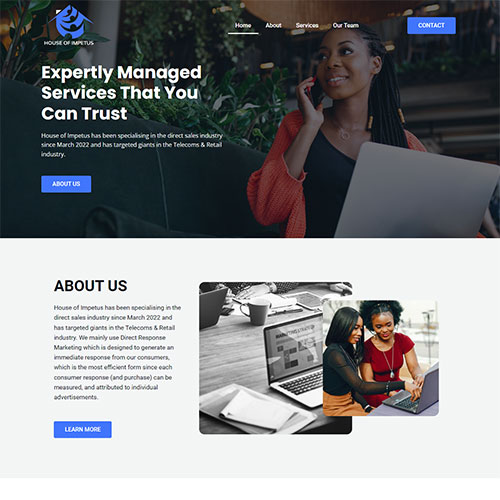The web page displayed features two horizontally stacked sections, each containing an image. 

In the top section, a Black woman with long braided hair is pictured, wearing an orange and black top. She holds a black cell phone to her ear while sitting in front of a laptop, which is seen from the back. The background includes some green plants on the left and a white text overlay that says, "Expertly manage services that you can trust." Beneath this slogan, there's additional white text that's too small to read, followed by a prominent blue button labeled "About Us."

The bottom section showcases an image on a white background. Here, two women are seated side by side, concentrating on an open notebook computer in front of them. To their left, the viewer can see another notebook depicted in black and white.

This descriptive composition highlights not just the visual elements but also the text details and layout design, providing context for the images presented.